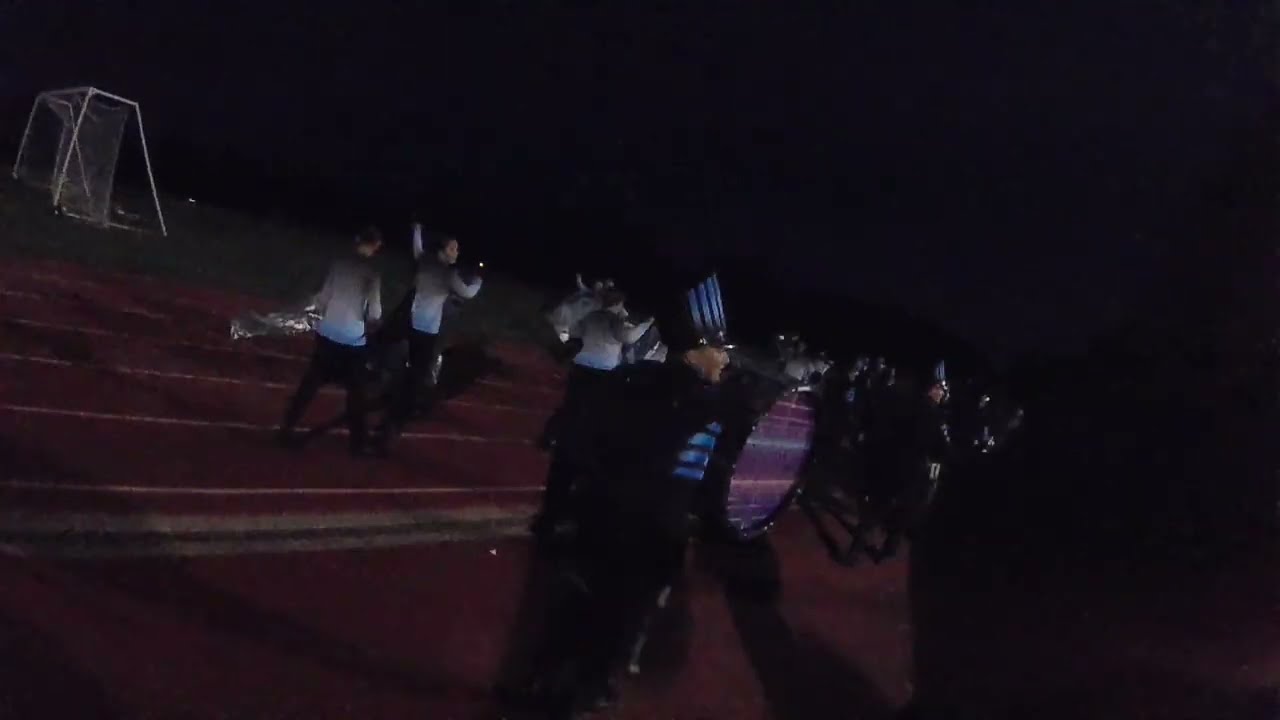This image, taken at night, depicts a high school marching band on a track and field area, shrouded in darkness that makes details sparse. The central focus is on a drummer, notable for his large drum strapped to his chest and his distinctive top hat featuring blue and black bars. His shirt mirrors the hat's design. Other band members are visible to his left, dressed in uniforms that blend from blue at the hips to white, then black at the shoulders. They are walking on a red track, with a soccer goal with a white bar and net visible in the upper left corner. The background is completely black, highlighting the dimly lit scene. The overall color palette of the image is dominated by very dark red, black, and flashes of blue, with some areas showing green grass in the middle of the track, indicating the school’s sports field under night conditions.